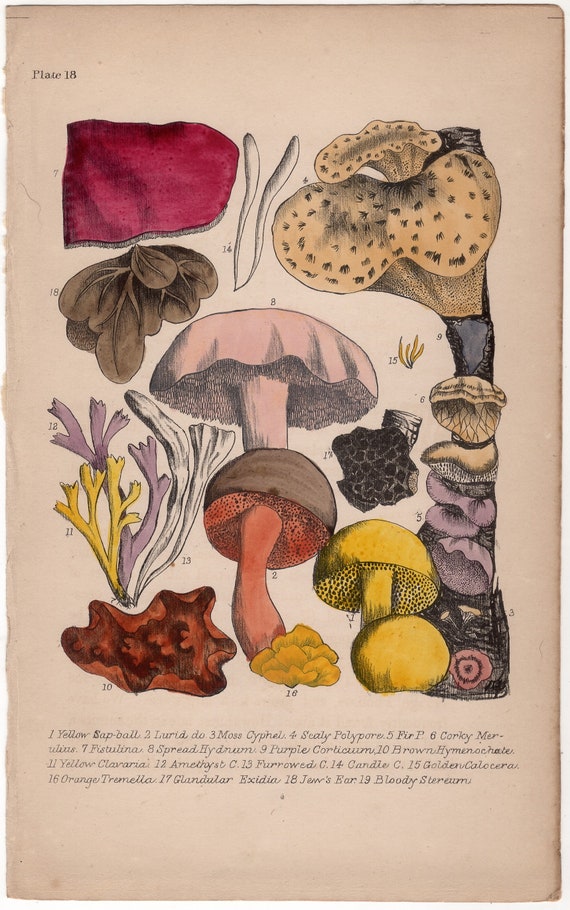The image depicts a color photograph of a worn and aged page, possibly torn from an old book, showcasing various types of mushrooms in the wild. The background of the page has a yellowish-tan hue, indicating its antiquated nature. At the top left corner, the text "Plate 18" is visible, labeling the collection. The central focus of the image is an array of meticulously illustrated and colored-in mushrooms in hues of red, pink, purple, yellow, orange, tan, and brown. Each mushroom is labeled below in small, somewhat unclear print. Although some of the names are difficult to decipher, they include titles like "Yellow Dapple Ball," "Lurid Dough," "Moth Stifles," "Feely Polypear," and "Purple Corticum." The detailed illustrations vividly capture the natural colors and diverse forms of fungus, creating a rich, botanical reference piece. Despite the aged quality and blurry text, the image stands as a fascinating display of wild mushrooms and their unique variations.